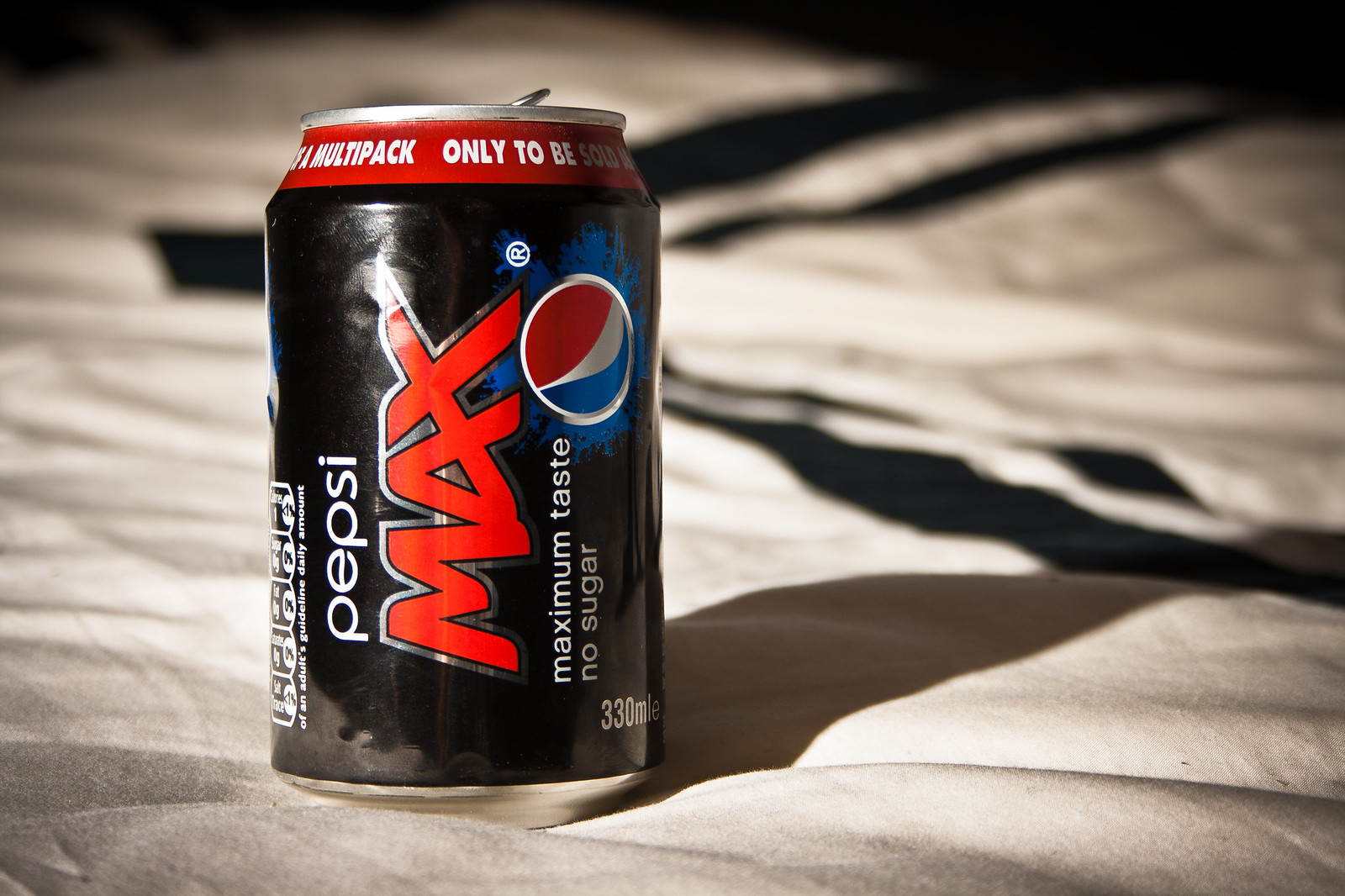This is a detailed photograph of a 12-ounce (330-milliliter) Pepsi Max can. The can predominantly features a black color scheme, diverging from the typical Pepsi blue, with striking red lettering for "Max" and accents around the Pepsi logo, which contains some typical blue elements. Clearly displayed on the can is the slogan "maximum taste, no sugar." The text on the can is oriented vertically. Near the top, a red band includes a partial warning in white letters indicating that the item is part of a multi-pack and cannot be sold individually. The can is situated on a white comforter with visible fabric texture and subtle waves, giving a sense of softness and slight crunchiness. In the background, there's a dark border on the comforter and diagonal shadows, adding depth to the photograph. The scene is well lit, emphasizing the details of both the can and the surrounding fabric.